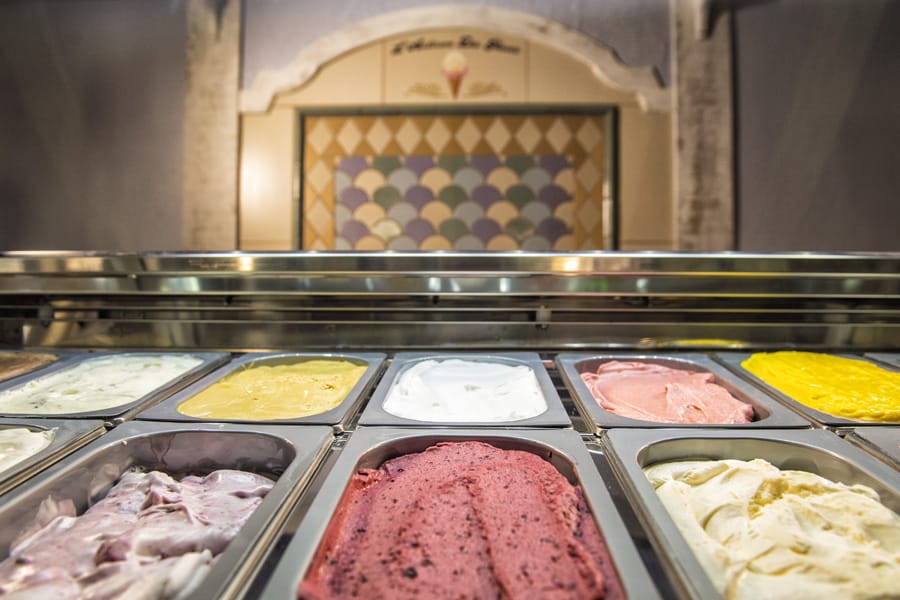This is a square, full-color, staged indoor photograph taken under artificial lighting. The image centers on an array of rectangular metal trays filled with a variety of vibrantly colored substances, likely ice creams or similar frozen desserts, arranged within what appears to be a display counter. The trays, which occupy the lower half of the photo, feature an assortment of flavors: on the far right is a vibrant yellow, followed by a pink, an off-white, another yellow, and a white. In the center is a striking red dessert with black specks, possibly strawberry-flavored. 

The metallic edge of the display counter partially covers the trays, which resemble those you might find in a restaurant or buffet setting. The close-up angle emphasizes the diverse colors and textures of the contents. The backdrop is blurred but discernible, featuring a creatively designed wall with a checkerboard and mosaic-like pattern, possibly evoking the appearance of ice cream scoops in colors like purple, bone-white, and green, enclosed in diamond shapes with gold trim. This whimsical decor reinforces the ice cream shop ambiance, making it a vibrant and inviting scene.